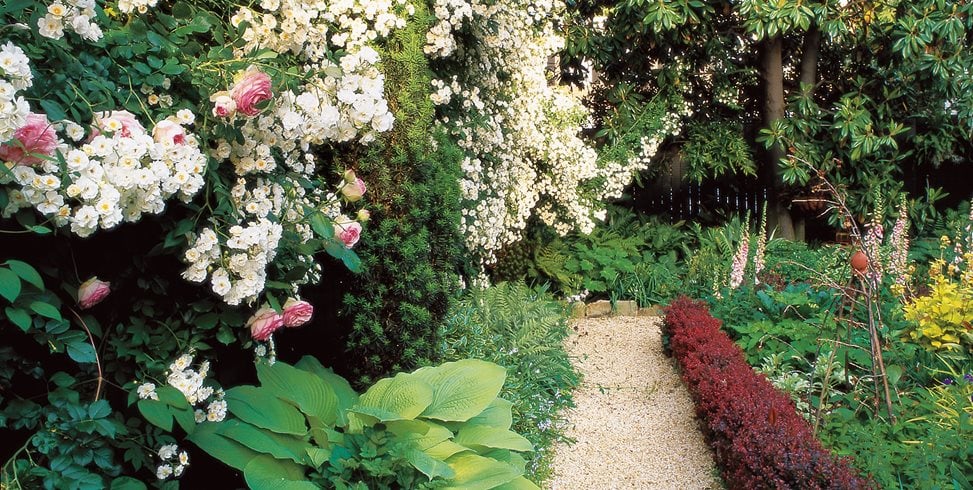This photograph captures a serene garden during the daytime, with the absence of direct sunlight suggesting an overcast sky. The image is in landscape orientation, showcasing a lush, blooming garden that emanates tranquility. A white pebble stone pathway runs through the center of the garden, inviting viewers to embark on a peaceful stroll. The pathway is bordered by short, maroon-colored barberry bushes, providing a striking contrast to the myriad of colors around it. To the left of the path, a large green-leaved hosta plant stands out, surrounded by a variety of green foliage and flowering shrubs. Prominent among these shrubs are clusters of white flowers with tiny yellow centers, alongside a sprinkling of delicate pink blooms.

In the background, taller trees with dark green canopies are interspersed with some adorned in white and pink flowers, adding height and depth to the scene. On the right side of the pathway, more green foliage flourishes, including vertical plants that resemble snapdragons and possibly a magnolia tree further back. A small bunch of yellow flowers peeks out from the far right corner, completing the vibrant and diverse floral tapestry. The presence of a dark fence in the distance underlines the backyard setting, making this garden not only beautiful but an intimate escape into nature's splendor.